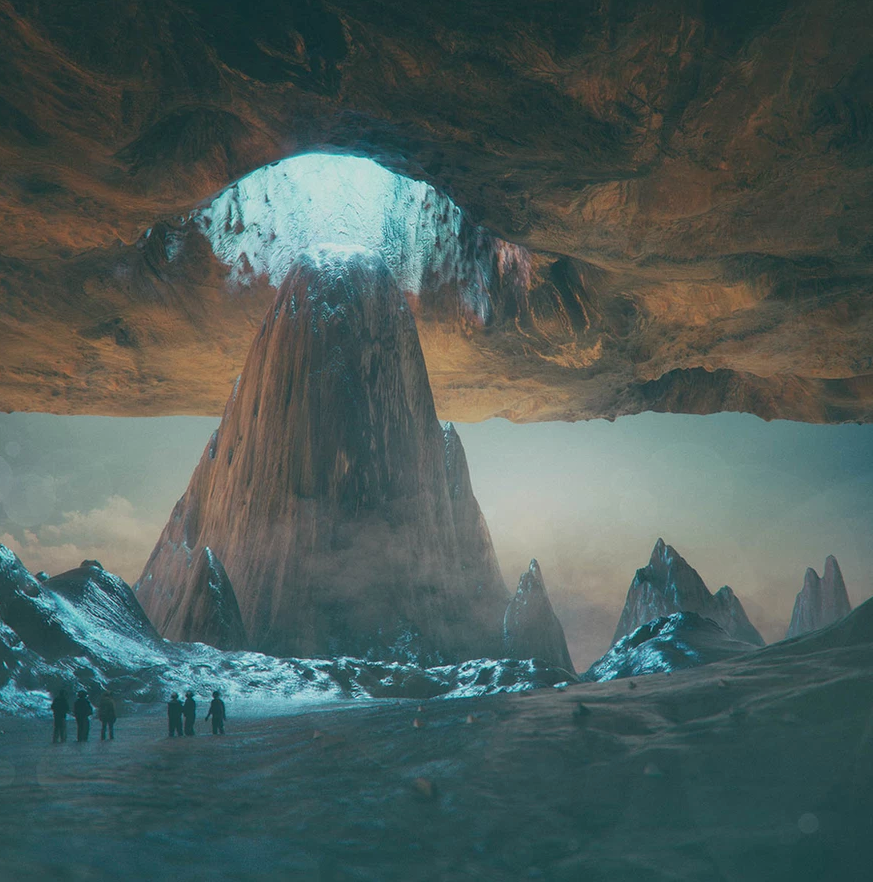In this fantastical digital image, six people are standing in two groups of three at the base of a towering mountain. The mountain is steep and narrow, capped with snow, and set within a wide expanse of land featuring a mix of brown and bluish hues. The scene is framed by a rocky surface above, creating an illusion reminiscent of "Journey to the Center of the Earth." At the very top of the mountain, there's a striking white hole emitting a bright light, suggesting an entry point to another world. This hole is positioned directly above the mountain peak with a backdrop of a gloomy, clouded sky, further enhancing the surreal and mystical atmosphere. The upper layer of the image is dominated by this rocky surface, which intriguingly replaces the sky, further emphasizing the fantasy element.